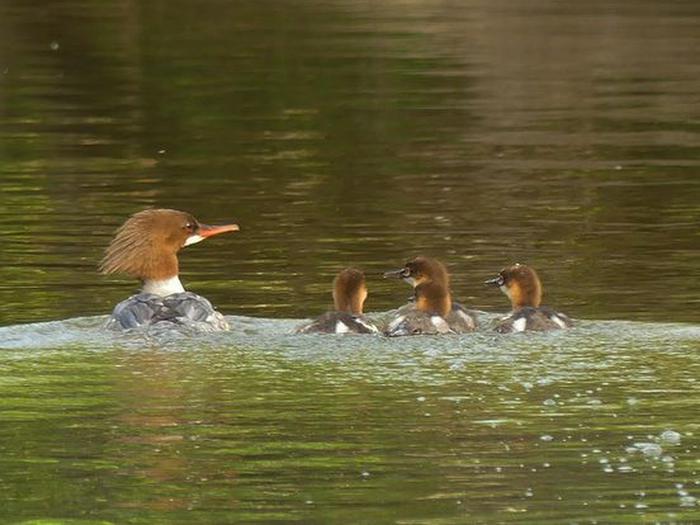This is a nature photograph capturing a serene scene of four ducks swimming in a pond with greenish-hued water, likely from algae or the reflection of surrounding trees. The central focus is a larger duck on the left, likely a parent, accompanied by three smaller ducks, presumably its offspring, swimming in a row to its right. The largest duck has distinctive features: an orange beak, brown feathers, a white neck, and spiky hair-like feathers at the back of its head, with the rest of its body submerged. The three smaller ducks mirror the adult's color pattern but have black beaks instead. The water is gently disturbed by their movement, creating bubbles and ripples, and the scene is bathed in sunlight, accentuating the ducks' various shades of brown, gray, and white feathers.